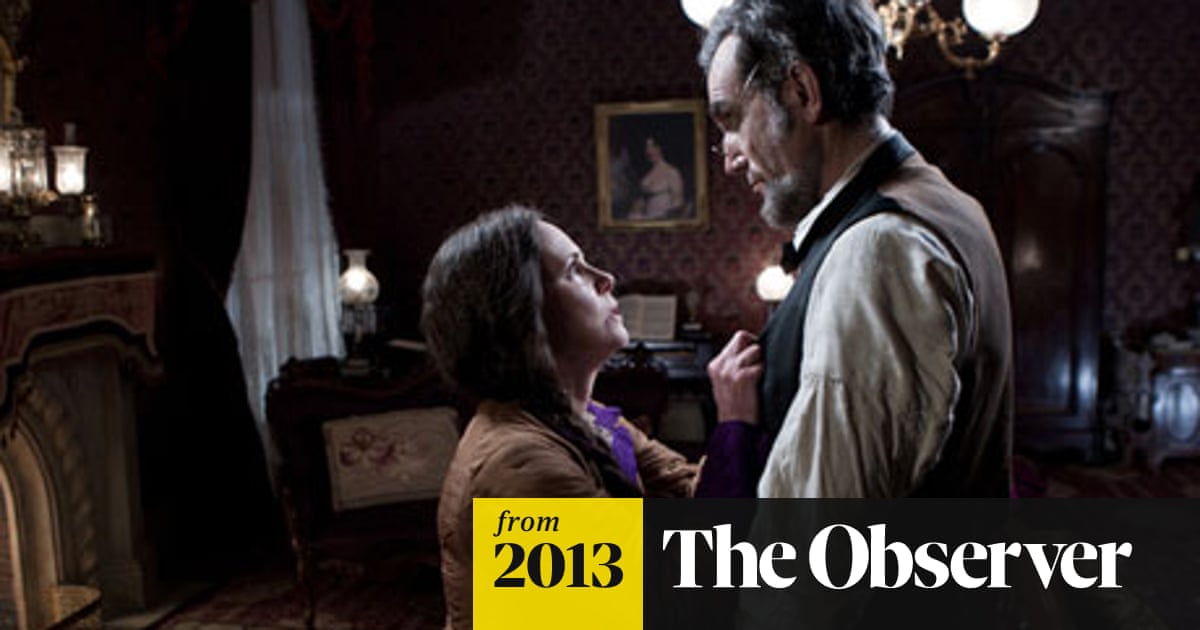The color photograph is a still from the 2013 movie "The Observer," featuring a scene with Sally Field and Daniel Day-Lewis, the latter portraying Abraham Lincoln. The two actors are the central focus, with Sally Field looking up at Daniel Day-Lewis, who is dressed as Lincoln in a white shirt, dark vest, and glasses. They are positioned in a detailed and historically styled parlor, which could belong to Mary Todd Lincoln, potentially even a room in the White House.

The room is richly adorned: 
- The backdrop features an ornate maroon wallpaper.
- Below it, there's a dark brown armoire.
- To the left, a window is draped in both sheers and curtains.
- A chandelier with globes hangs from the ceiling.
- Lit oil lanterns are spread throughout the scene, including along the fireplace and on a table, enhancing the room's warm, intimate ambiance.
- A blurred portrait of a lady can be seen in the background above a piano.

Overall, this image captures a poignant moment between the two characters amidst a classic and elaborately decorated historical setting.